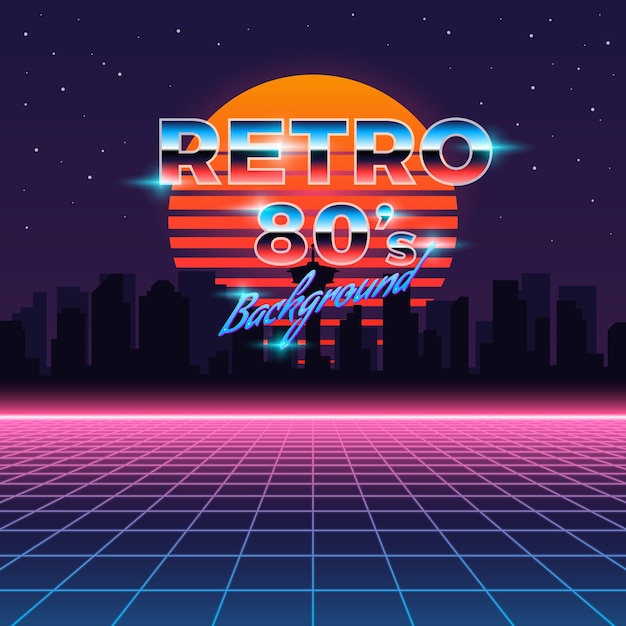The image is a vibrant retro 80s-themed advertisement set against a dark, starry night sky filled with small white dots representing stars. Dominating the scene is an iconic sun design positioned at the center, characterized by its horizontal lines that transition from a vivid orange at the top to a rich red at the bottom. Above the sun, in bold, capitalized letters, is the word "RETRO," featuring a gradient that moves from blue at the top through white and black, ending in red at the bottom. Below "RETRO" is the term "80s" in a similar gradient style, followed by the word "BACKGROUND" in italicized letters.

The lower portion of the image features a black silhouette of tall skyscrapers, framed by a bright neon pink horizontal line extending across the image. Below this, the foreground introduces a gridded pattern resembling a digital floor, composed of blue and pink colors with intersecting white lines, giving a sense of perspective and depth. The entire scene exudes a nostalgic 80s vibe through its use of bold colors, geometric shapes, and retro-futuristic aesthetic.